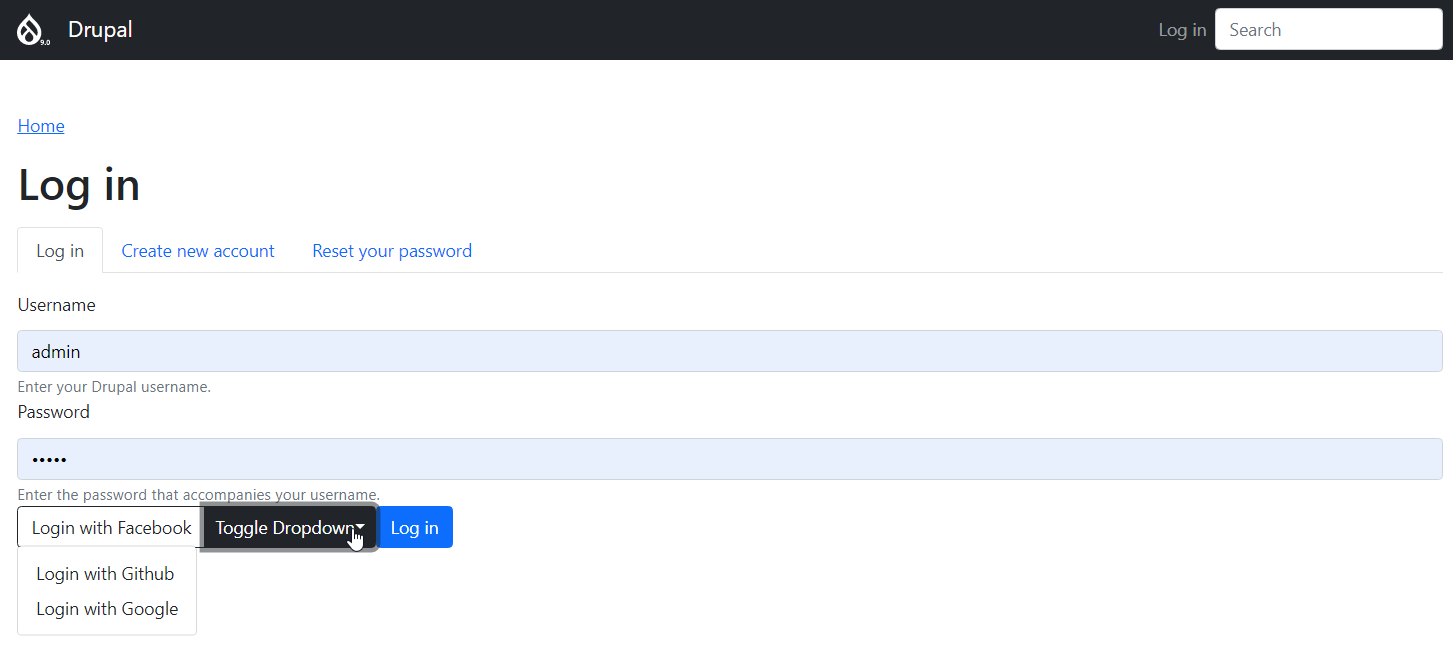The image is a screenshot of the login page for the Drupal website. At the top of the page, a black bar spans the entire width of the screen. On the left side of this bar, the word "Drupal" is prominently displayed in white font. Accompanying the text is a logo that resembles a leaf or a teardrop with intricate markings inside, also rendered in white.

On the right-hand side of the black bar, there is a login button, followed by a search bar positioned to its right. Directly below the black bar is a blank white space that acts as a line separator.

The main content of the page begins below this white space. On the left, the word "Home" appears in blue, underlined, and starting with a capital "H." To the right of this, in slightly larger black font, is the text "Log in," with both words capitalized appropriately.

Beneath this heading, there are three tabs presented horizontally: "Log in," "Create new account," and "Reset your password," with the "Log in" tab currently selected. Within the "Log in" tab, the username field is visible, pre-filled with the text "admin."